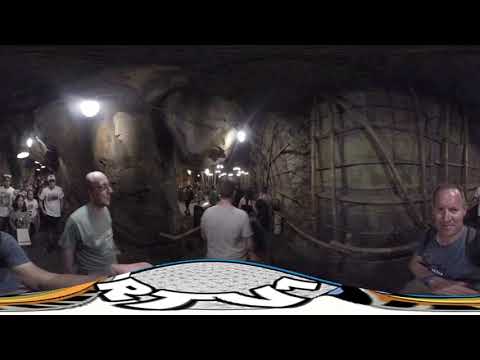Captured in a dim, grayish-brown, cavernous setting reminiscent of an underground tunnel or perhaps the Raiders of the Lost Ark ride at Disneyland, this blurred photograph showcases a bustling interior space that could be a dungeon or catacomb-like structure. The setting features rugged stone walls supported by rebar and adorned with ropes, giving it a man-made cave appearance. Toward the center of the image stands a man in a white t-shirt with his back to the camera, seemingly entering through an open archway that leads to a long, dimly lit hallway filled with numerous overhead lights and people.

In the foreground, on the right side of the image, a man in a gray t-shirt smiles at the camera. He is an older, bald, clean-shaven gentleman and appears to be seated at a registration table, which has "RTV1" curved lettering on its white top. To his left, another similar-looking man, also in a gray t-shirt, stands or sits, facing slightly right, perhaps observing the corridor. Additionally, a third man, partially visible on the far left edge of the picture, extends his right arm, resting it on the table.

The left side of the image reveals a corridor bustling with people entering the space, illuminated by more overhead lights. The ambiance is dark and mysterious, giving an impression of an event set in a cavernous, underground labyrinth.